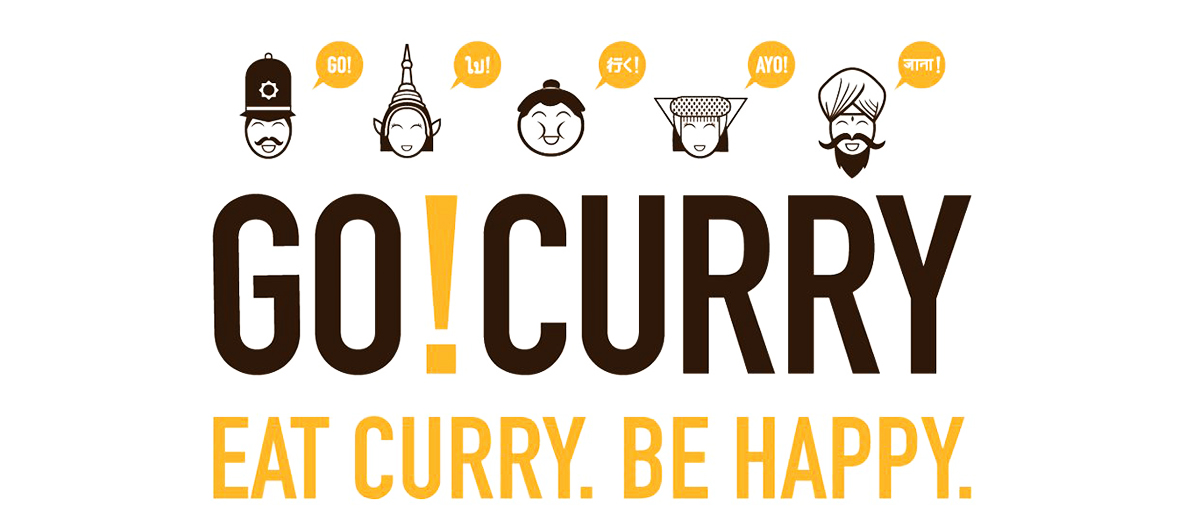The image features a simple graphic poster with a white background advertising curry. At the center, the large bold black letters "GO" are followed by a gold exclamation mark, and to the right, it reads "CURRY" in the same large black lettering. Below this, the vibrant gold and orange text states "EAT CURRY. BE HAPPY."

At the top of the poster, there are five different character illustrations, each enclosed in orange speech bubbles with different phrases. From left to right:

1. A character resembling an English bobby guard with a tall, rounded black helmet and a black mustache, with a speech bubble saying "GO!"
2. A small, Asian-looking character with a hat resembling a temple spire, speaking in unreadable Asian script.
3. A round-faced individual with dark hair styled into a bun or top knot, saying something in Chinese letters.
4. A female character, likely of Japanese or Korean origin, with black hair and a speech bubble containing the phrase "AYO!"
5. A monk-like figure with long dark hair, a beard, and a mustache, with the speech bubble showing Asian script. 

The poster uses shades of brown and orange, combining textual elements with detailed, cartoonish character drawings to create a lively and inviting advertisement.